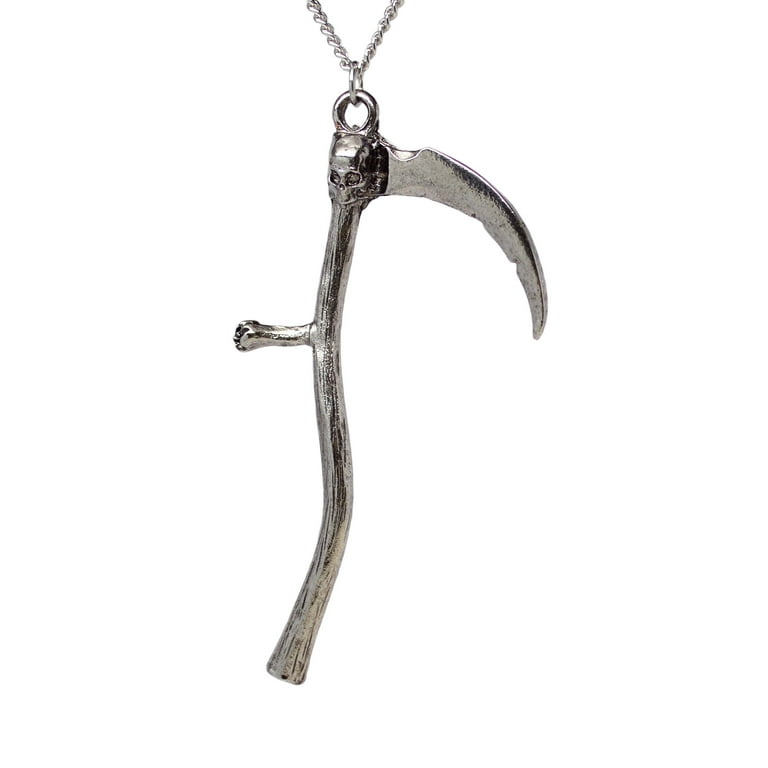The image is a close-up photograph of a silver necklace against a completely white background. The top of the chain is visible, cascading into two intertwined rings that suspend a singular charm in the shape of a scythe. The scythe, detailed in silver, features a curved handle with a protruding hand grip, mimicking a wooden texture. At the top of the scythe, a small, intricately crafted skull is placed where the blade meets the handle. The scythe’s blade, extending from the right side of the skull, is curved and notched, suggesting a sense of wear or damage. The charm, vivid and striking, evokes imagery of the Grim Reaper's iconic tool, adding a dark, gothic allure to the delicate piece of jewelry.